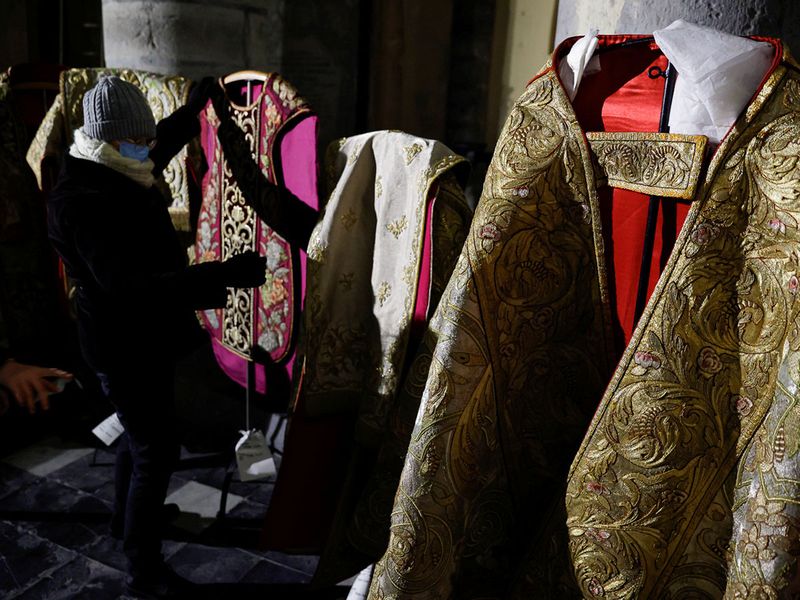In this detailed indoor photograph, we see a collection of ornate and beautiful clothing items displayed on wooden stands. The item closest to us on the right is a striking jacket with a golden exterior adorned with intricate floral or emblematic designs, and a rich red interior. Moving leftward, there's a vibrant hot pink garment with elaborate designs running down its center and gold trims, adding to its magnificence. Further left, a white and gold vestment or poncho stands out for its elegant simplicity.

Inspecting these garments is a person dressed in a black coat, black gloves, dark pants, and dark shoes. The individual is wearing a gray wool beanie, a blue face mask, and a light-colored scarf draped around their neck. They appear to be examining the pink garment closely, with their left hand holding up part of the fabric. Their cautious demeanor is emphasized by the protective face mask and the careful way they handle the clothing, suggesting an appreciation for the craft and beauty of these items. Glasses add a thoughtful touch to their appearance. 

The overall atmosphere of the image speaks to a quiet admiration of the ornate and beautifully detailed garments prominently displayed.